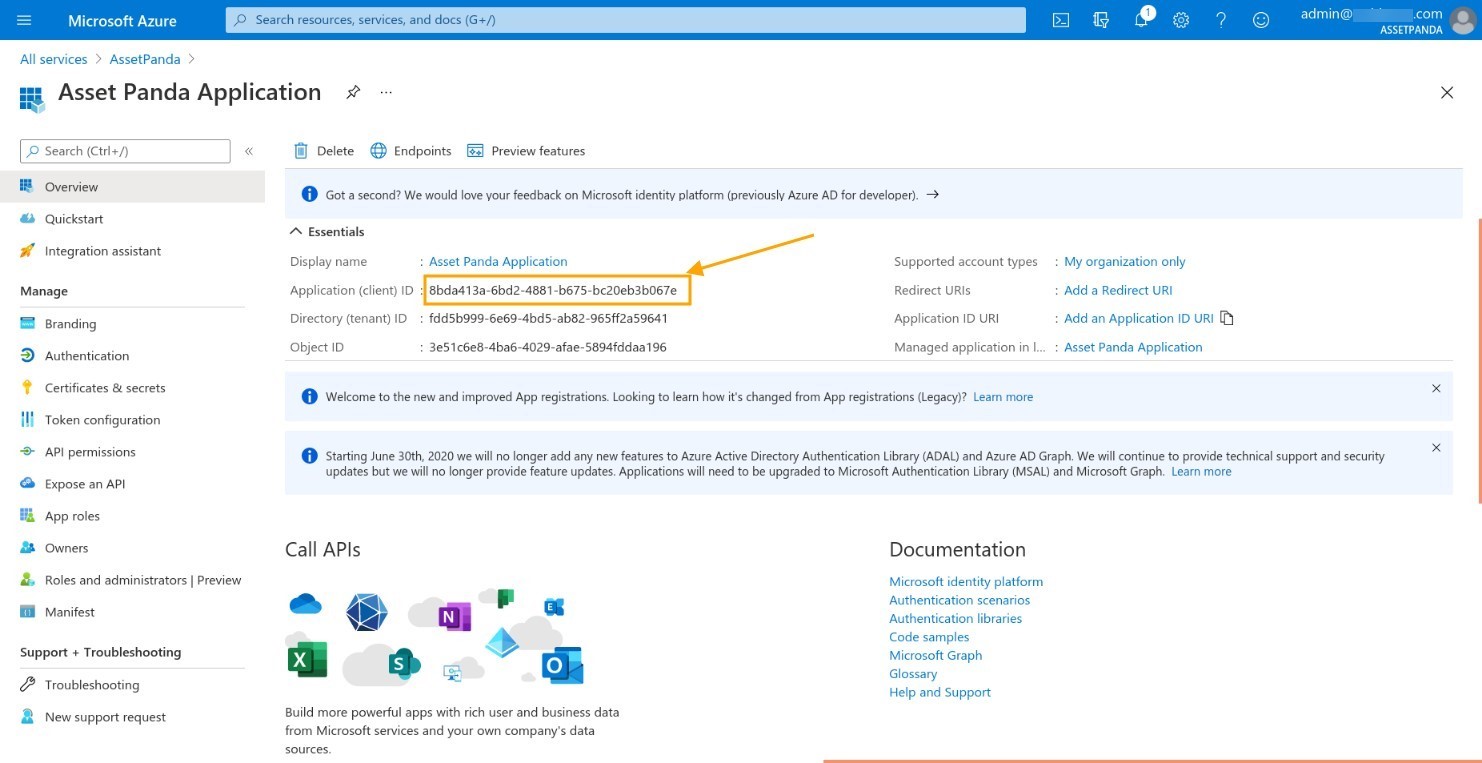In this image, a screenshot of a Microsoft Azure settings page is meticulously detailed. Dominating the top left corner is the "Microsoft Azure" label in small white text, indicating the specific platform. A dark blue navigation bar extends across the top of the screen, featuring a light blue search bar with black text centrally positioned. To the right of the search bar are several icons in white, including a settings icon, a question mark for help, and a notification bell symbol.

Beneath this navigation bar is a clean, white background forming the main part of the webpage. Along the left side, a vertical menu displays various tabs or buttons in small black text, each accompanied by an adjacent logo. These options include "Overview," "Quickstart," "Branding," "Authentication," "Certificates & secrets," and "Token configuration." 

On the right side of the page, a list of API-related information is presented. Long alphanumeric strings, representing IDs, are visible and are categorized as documentation IDs, directory IDs, and application IDs. The layout and the detailed options indicate a complex and comprehensive settings interface designed for detailed configuration and management within Microsoft's Azure platform.